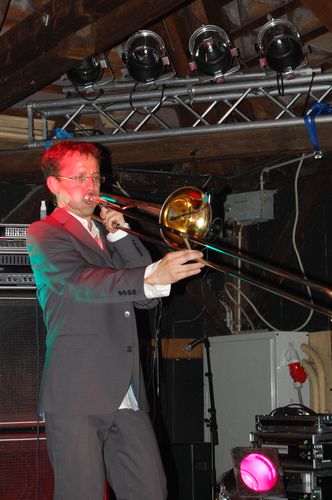In this image, a middle-aged white man is on stage, intensely playing a trombone with his cheeks puffed out as he blows into the instrument, extending it outward. He faces towards the right side of the photograph, seemingly ignoring the photographer, which allows a focused view of his expression and posture. Dressed in a dark gray suit with matching pants, the ensemble is accented by black and white buttons and paired with a white collared shirt and what looks like a red tie tucked into his collar. He wears thin, circular glasses and has brown hair, which appears to be thinning, although it gets a reddish tint from a stage light above his head.

The stage setup includes a metal rod above him, holding four stage lights pointed in various directions, although these lights do not appear to be actively illuminating the scene. Additional reflections from green, yellow, and red lights gleam off the trombone and add a greenish hue to his shoulder. This lighting setup creates interesting highlights and shadows, contributing to the photograph's dynamic lighting.

In the background, behind the man, there is a large speaker likely being used to project the music to the crowd and some electrical wires and a box visible. A distinct purplish-pink spotlight casts a subtle glow from the lower right-hand corner of the image, adding a touch of color to the otherwise neutral tones of the stage surroundings. Despite the complexity of the stage equipment and lighting, the focus remains on the man's dedicated performance.